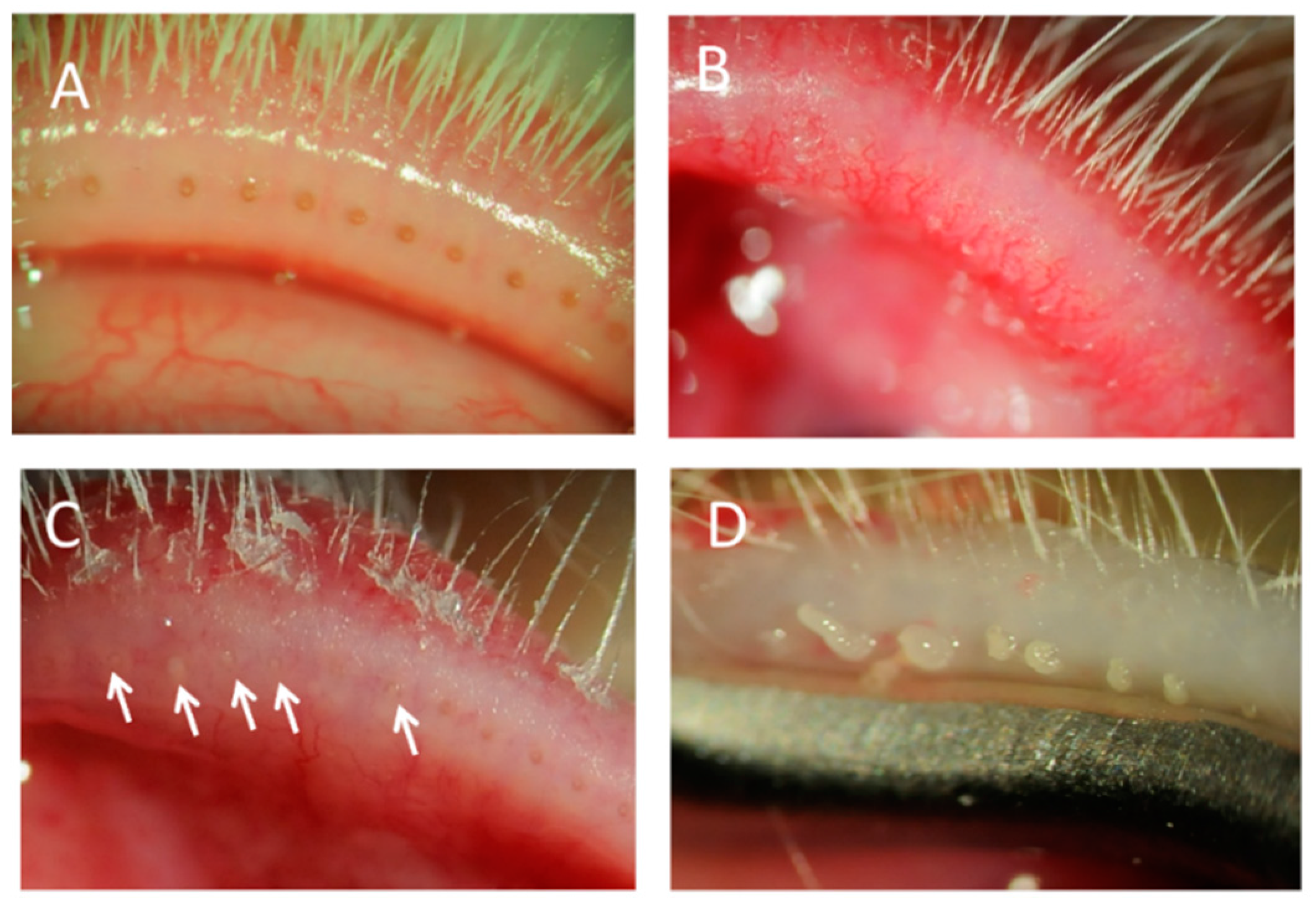The image is a large rectangular collage consisting of four quadrants (A, B, C, D), each capturing an extremely close-up view of an eyelid that appears to be under a microscope. In each quadrant, you can distinctly see the white, almost clear eyelashes protruding from the eyelids. The images reveal various conditions affecting the eyelids, such as redness, inflammation, and what appears to be pus or small dots. The capillaries with blood flow are also visible in these high-magnification shots.

- **Quadrant A (upper left)**: Displays the inside of an eyelid with visible small hairs emerging and hints of the upper part of the eye. 
- **Quadrant B (upper right)**: Shows an inflamed, red eyelid with protruding hairs and a part of the eyeball.
- **Quadrant C (lower left)**: Features an eyelid that appears wide open with red coloration, marked by white arrows pointing to specific spots. The hairs look messy and fragmented, with a blurred section of the eyeball underneath.
- **Quadrant D (lower right)**: Depicts a more tan-colored eyelid, with apparent tears or droplets on it, just above the eyelid line, alongside a black line marking the lower eyelid area.

Each quadrant potentially suggests signs of eyelid conditions or diseases, possibly involving mites or other irritants, emphasized by the enhanced microscopic perspective. The imagery, though blurred, portrays a detailed and somewhat eerie examination of eyelid anatomy, which could be of an animal or a distorted representation of a human eyelid.